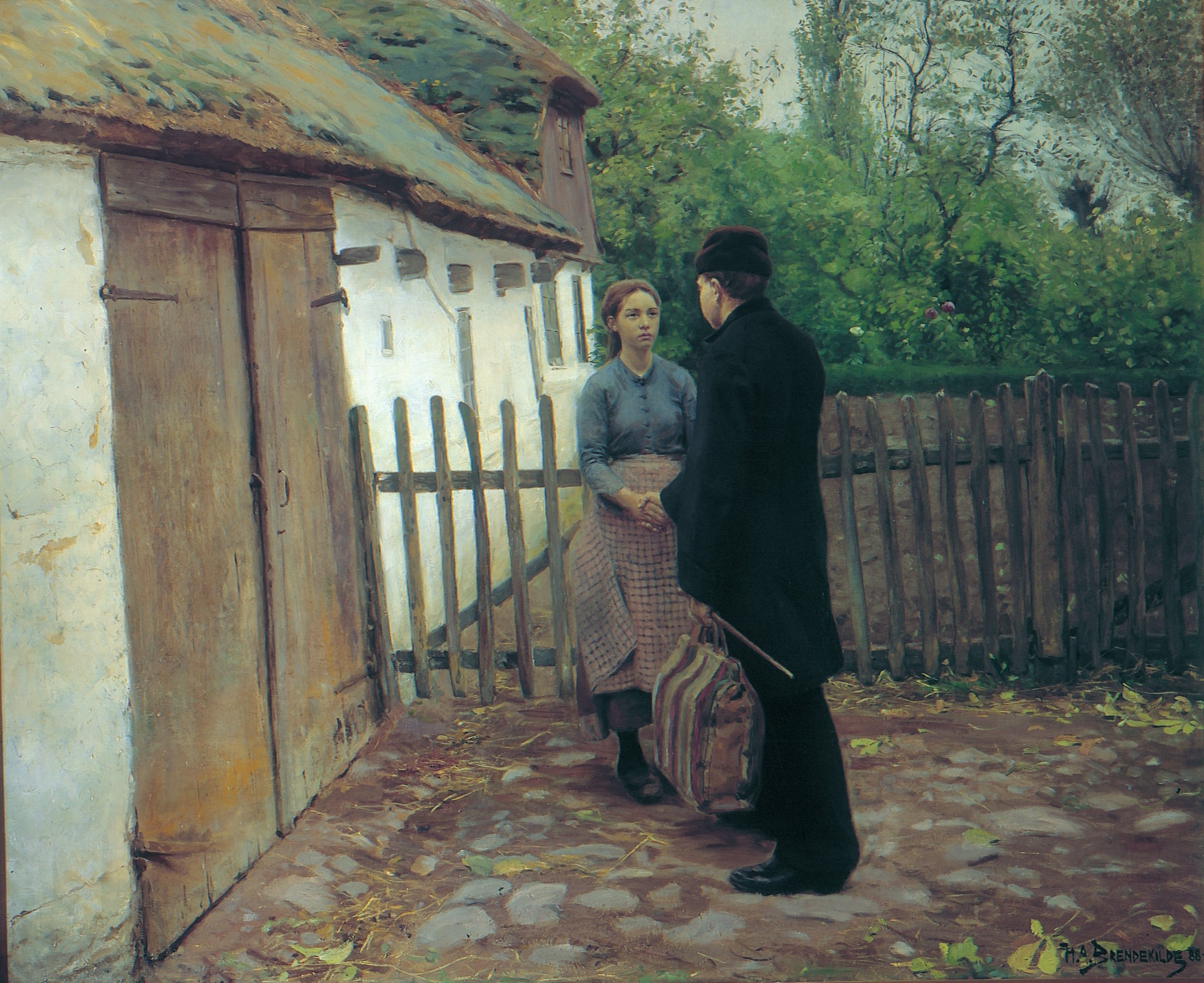In this hyper-realistic painting, reminiscent of a photograph, a poignant scene captures a man and a woman engaged in a handshake in what appears to be a late afternoon setting. The backdrop consists of thick, dense trees under a grayish sky, visible only in the upper right-hand corner. Dominating the right side of the painting is a rocky ground interspersed with patches of brown dirt and gray rocks. To the left stands a rustic, white-walled house with a brown roof, seemingly adorned with green moss. A brown door on the left side of the house opens to a simple, rustic horizontal-wood fence.

The man, dressed entirely in black with a hat that resembles a Russian style, carries a suitcase and a cane. His back is to us, obscuring his face. Opposite him, a woman in a blue dress and apron gazes at him with an expression tinged with sadness. Their attire suggests a period from either colonial days or the 1950s. The simplicity and earthy tones of the scene, combined with the detailed portrayal of their attire and somber interaction, evoke a deep sense of time and place.